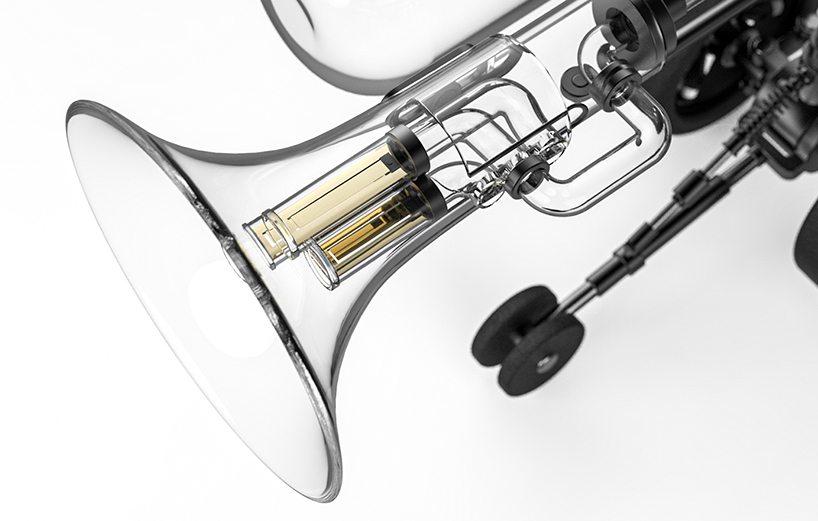The image depicts a close-up of a mechanical or scientific apparatus set against a plain, bright white background. Central to the device is a large, trumpet-shaped glass component that resembles a funnel or horn. The glass is clear but features a silver coating near its base. Within this glass funnel are two smaller cylindrical vials; the upper vial contains a light, more fluorescent yellow material, while the lower vial holds a darker, vibrant yellow substance. Surrounding and connecting to this glass structure are various metal parts, including springs, pumps, and tubes, suggesting a complex system intended for movement or fluid transfer. To the right, the apparatus includes additional silver metallic sections, all leading down to a pair of black wheels connected by a steel arm, indicating a potential for mechanical operation or movement. Despite the detailed components and intricate design, the exact function of the device remains unclear.